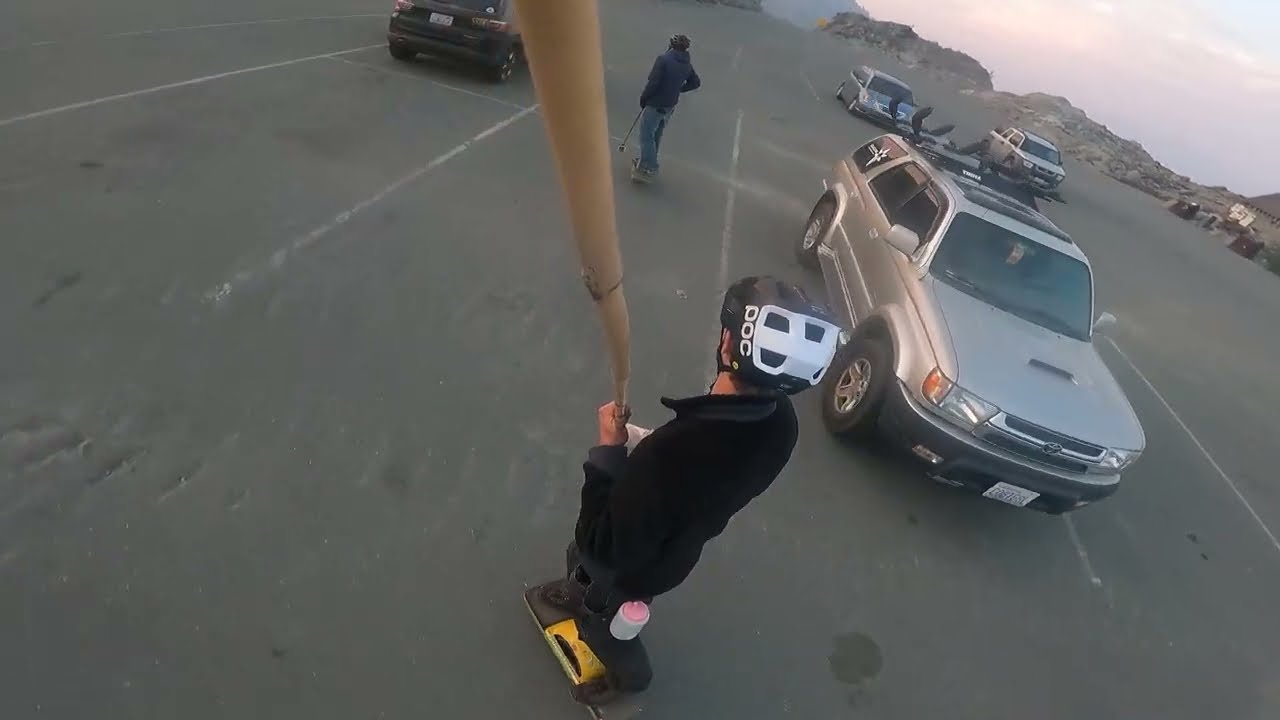In this image, a person dressed in black clothes and wearing a distinctive white helmet, bearing the POC logo, is skateboarding in a large parking lot while taking a selfie with a selfie stick. The selfie stick is extended behind them, capturing the scene from an unusual angle. The setting is during the day, under a sky filled with clouds that appear slightly reddish. Multiple cars are parked in the lot, including a silver SUV, a silver truck, a gray car, and another black SUV. The light gray asphalt ground features faded parking spaces and a dumpster off to the side. Another person, also on a skateboard, is visible in front of the main subject. Additionally, rocky structures can be seen in the distance.